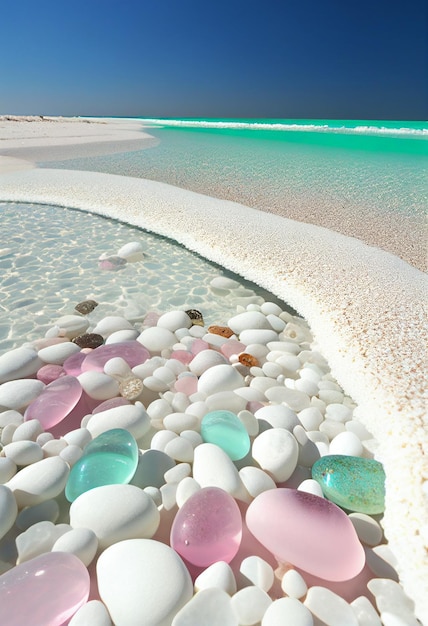This striking image, likely enhanced by hyper-realistic AI, captures an outdoor beach scene with vivid detail. At the top, the sky transitions from a dark blue, almost purple hue on the right, to a lighter blue on the left, unmarred by clouds. Below, a neon sea green ocean, accentuated by a uniform white line of waves, dominates the upper portion of the scene as it approaches the shoreline. 

In the middle and toward the bottom of the image, light, almost white sand stretches out, framing a small, stone-paved pool of water. This pool contains an array of perfectly smooth pebbles—most predominantly pure white but also featuring striking pinks, teals, and a few small red and brown stones. These pastel-colored stones, reflecting the light beautifully, almost resemble opals and create an ethereal blend of colors and textures. This picturesque foreground is seamlessly connected to the shallow, greenish beach water, providing a captivating and serene coastal vista.